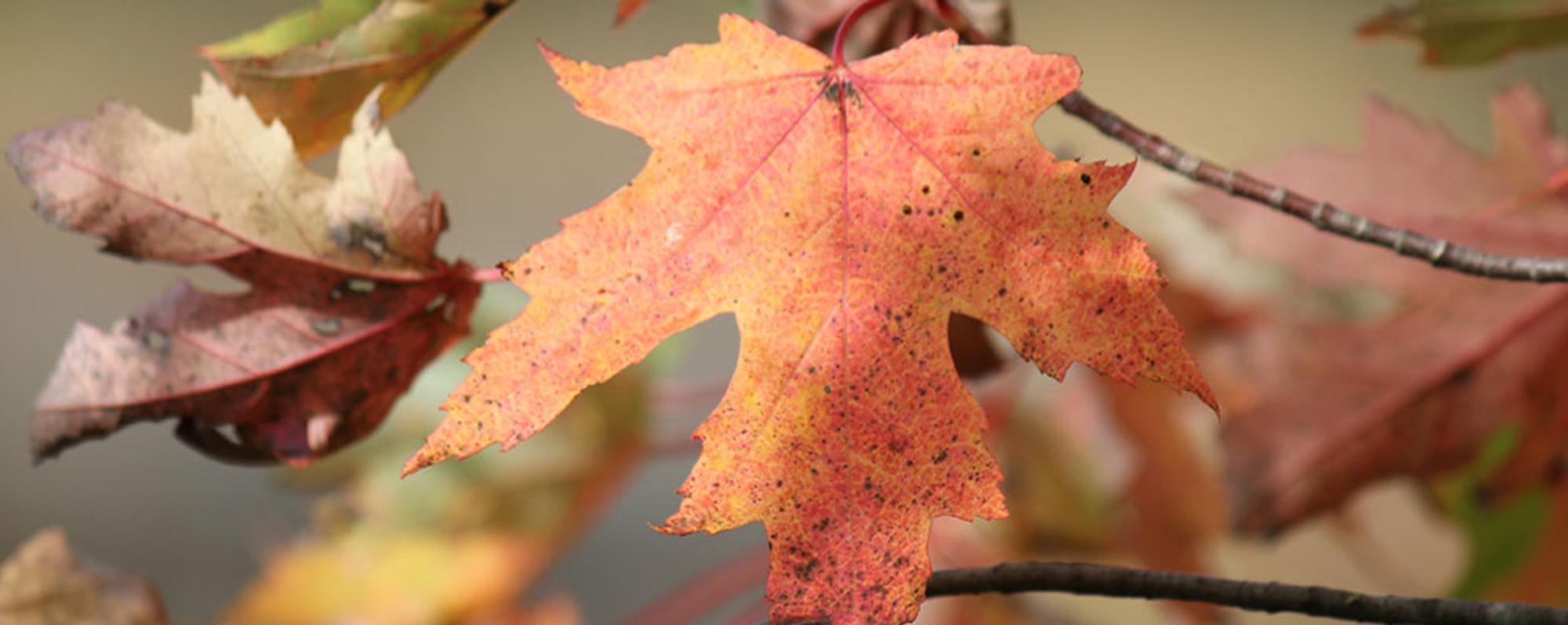This image captures a close-up of a vivid maple leaf centered in the frame, showcasing its intricate autumn colors of orange and light reddish-pink with visible red veins and black spots. The leaf's stem extends from the top, and its lower point stretches out of the image's frame. Surrounding this central leaf, the background features a light brown or tan hue adorned with blurred maple leaves in shades of light brownish-red, yellow, and green, indicating the scene's seasonality. To the left, several leaves are visible, including a decaying one with black spots and holes, a greenish-yellow leaf at the top, and a yellow leaf at the bottom near a partial brown leaf in the lower left corner. Two thin branches traverse the upper right quadrant of the image, adding depth to the composition. The overall outdoor setting, coupled with the various stages of leaf decay and autumn shades, suggests this photograph might be suited for educational purposes or as a detailed representation of fall foliage taken by an amateur enthusiast.